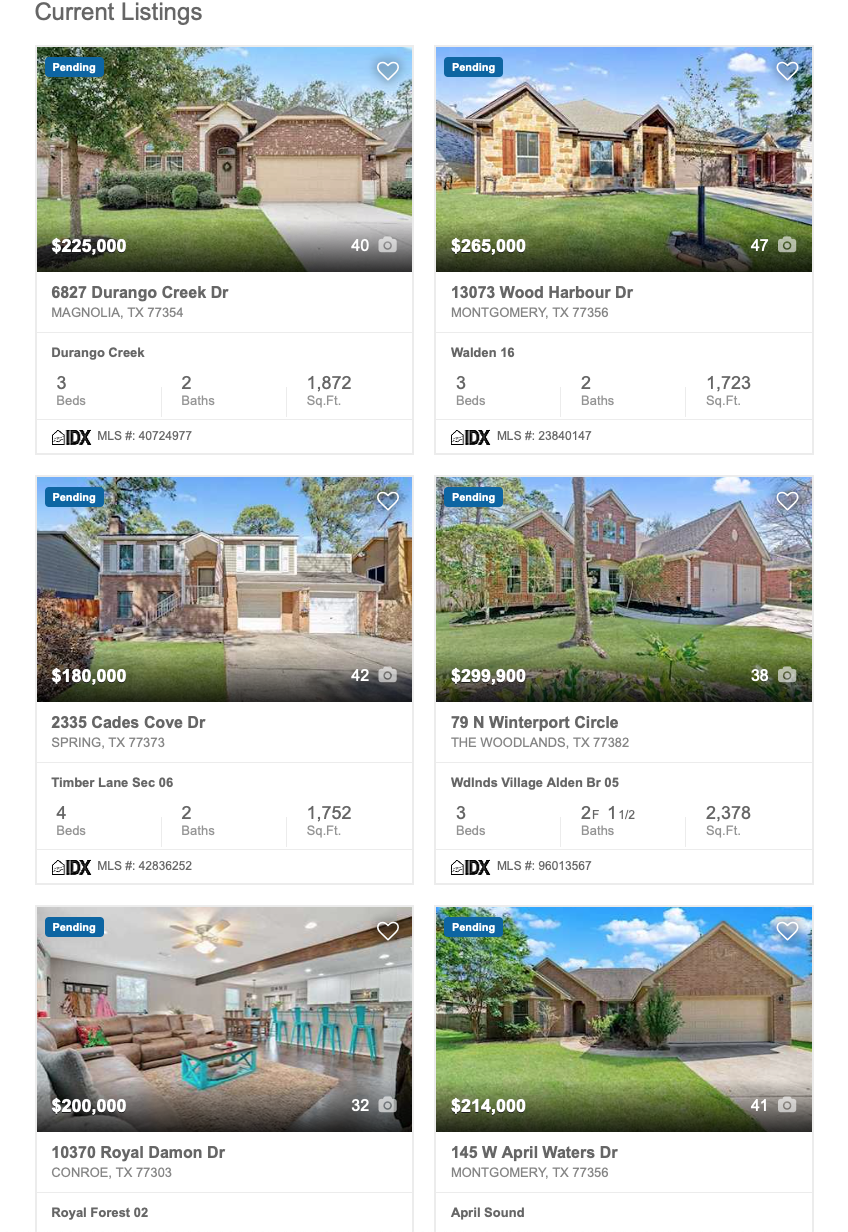### Detailed Property Listings

**Image Description:**
The image features a white background with detailed descriptions of current property listings. The properties are listed as follows:

1. **Top Left Corner:**
   - Text: "Current Listings" in gray.
   
2. **First Property:**
   - Status: Pending
   - Image: Shows a house with a green lawn and gray driveway.
   - Price: $225,000
   - Views: 40 (indicated by a camera icon)
   - Address: 6827 Durango Creek Drive, Magnolia, Texas, 77354
   - Description: Durango Creek, 3 bed, 2 bath, 1,872 square feet.
   - MLS Number: 40724977
   - Realtor Logo: Present
   
3. **Second Property:**
   - Status: Pending
   - Image: Shows a house with green grass, one tree in the front, blue sky, and gray driveway.
   - Price: $265,047
   - Views: 47 (indicated by a camera icon)
   - Address: 13073 Wood Harbor Drive, Montgomery, Texas, 77356
   - Description: Walden 16, 3 bed, 2 bath, 1,723 square feet.
   - MLS Number: 23840147

4. **Third Property:**
   - Status: Pending
   - Image: Shows a house with a blue sky, gray concrete driveway, green grass, windows, and brick exterior.
   - Price: $180,042
   - Views: Indicated by a gray clock
   - Address: 2335 Cadiz Cove Drive, Spring, Texas, 77373
   - Description: Timber Lane Sec 06, 4 bed, 2 bath, 1,752 square feet.
   - MLS Number: 42838252

5. **Fourth Property:**
   - Status: Pending
   - Image: Shows a large tree in the middle, green grass, gray driveway, and blue sky.
   - Price: $299,938
   - Views: Indicated by a gray camera icon
   - Address: 79 N Winterport Circle, The Woodlands, Texas, 77382
   - Description: WDINDS Village, Alden, 3 bed, 2 full baths, 1 half bath, 2,378 square feet.
   - MLS Number: 96013567

6. **Fifth Property:**
   - Status: Pending
   - Image: Interior view with a white ceiling, white light, brown furniture, brown carpet, gray walls, and teal-colored seats by the bar.
   - Price: $200,000
   - Views: 32 (indicated by a camera icon)
   - Address: 10370 Royal Damon Drive, Conroe, Texas, 77303
   - Description: Royal Forest 02

7. **Sixth Property:**
   - Status: Pending
   - Image: Shows a house with green grass, gray driveway, off-white garage door, red brick exterior, and green tree to the left with some bushes in the center.
   - Price: $214,041
   - Views: Indicated by a camera icon
   - Address: 145 W April Waters Drive, Montgomery, Texas, 77356
   - Description: April Sound

Each property also features a gray and white outlined heart icon at the top right corner, denoting it is a favorite or watched property.